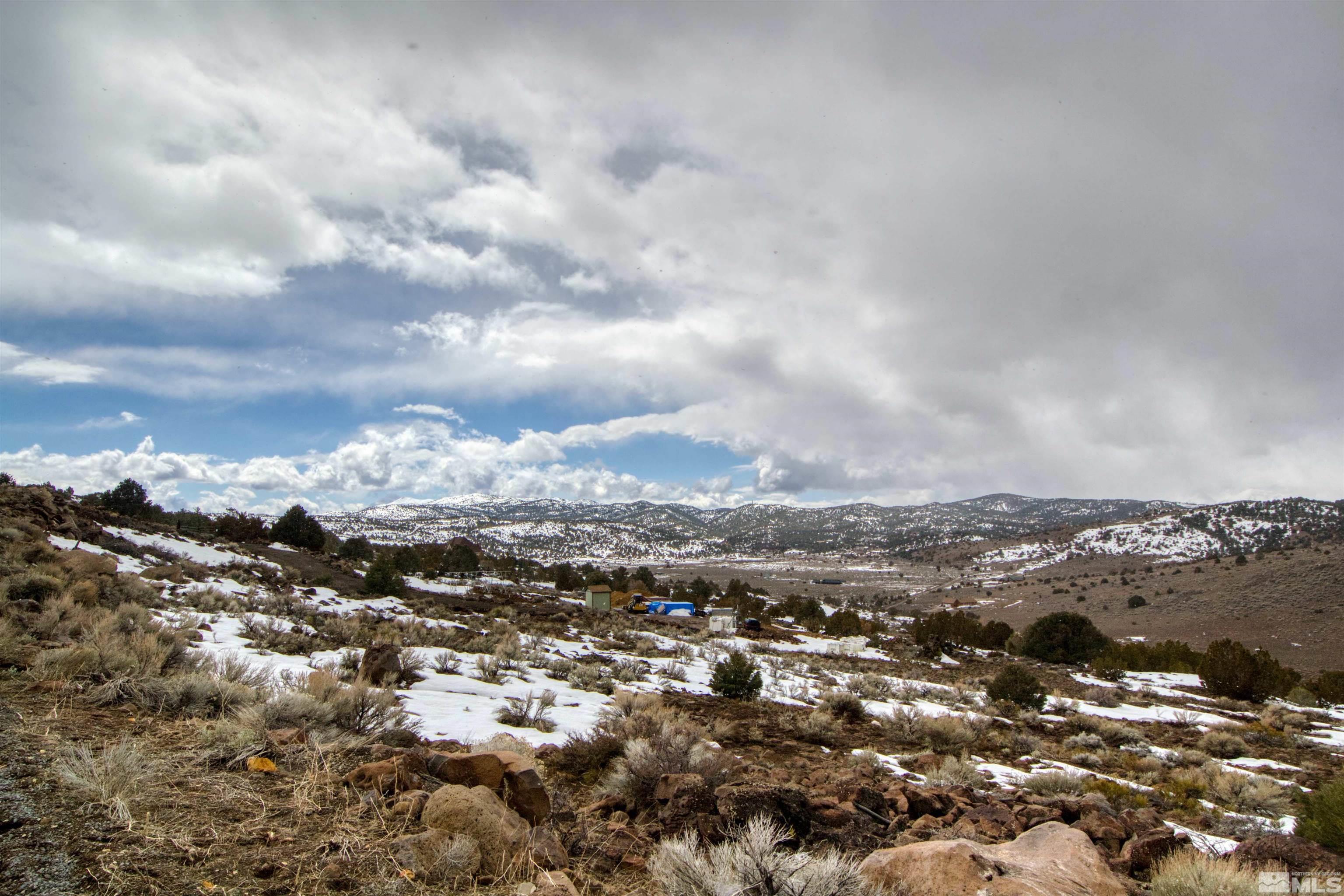This photograph captures a mountain landscape in winter. The bottom half of the image features a brown, sloping hill from left to right, with patches of snow and tufts of beige grasses, alongside dark green silhouettes of large bushes scattered across the slope. Further right, there's another hill partially covered in snow, descending leftwards. In the center of the frame, distant, bluish-brown mountains with scattered snow create a majestic horizon line. Above this horizon, the sky is predominantly cloudy, with thick gray clouds dominating the right side and patches of blue sky mixed with silver and white clouds on the left.

In the very center of the image, there is a collection of small buildings and objects, possibly part of a campsite or outpost. The buildings include a small olive shack with a reddish-brown pointed roof on the left, a nearly hidden yellow heavy machine, a blue structure covered in a blue tarp, and a small white rectangular object to the right. Sparse snow covers parts of the foreground, allowing the shrubs and plants to protrude from the wintry scene.